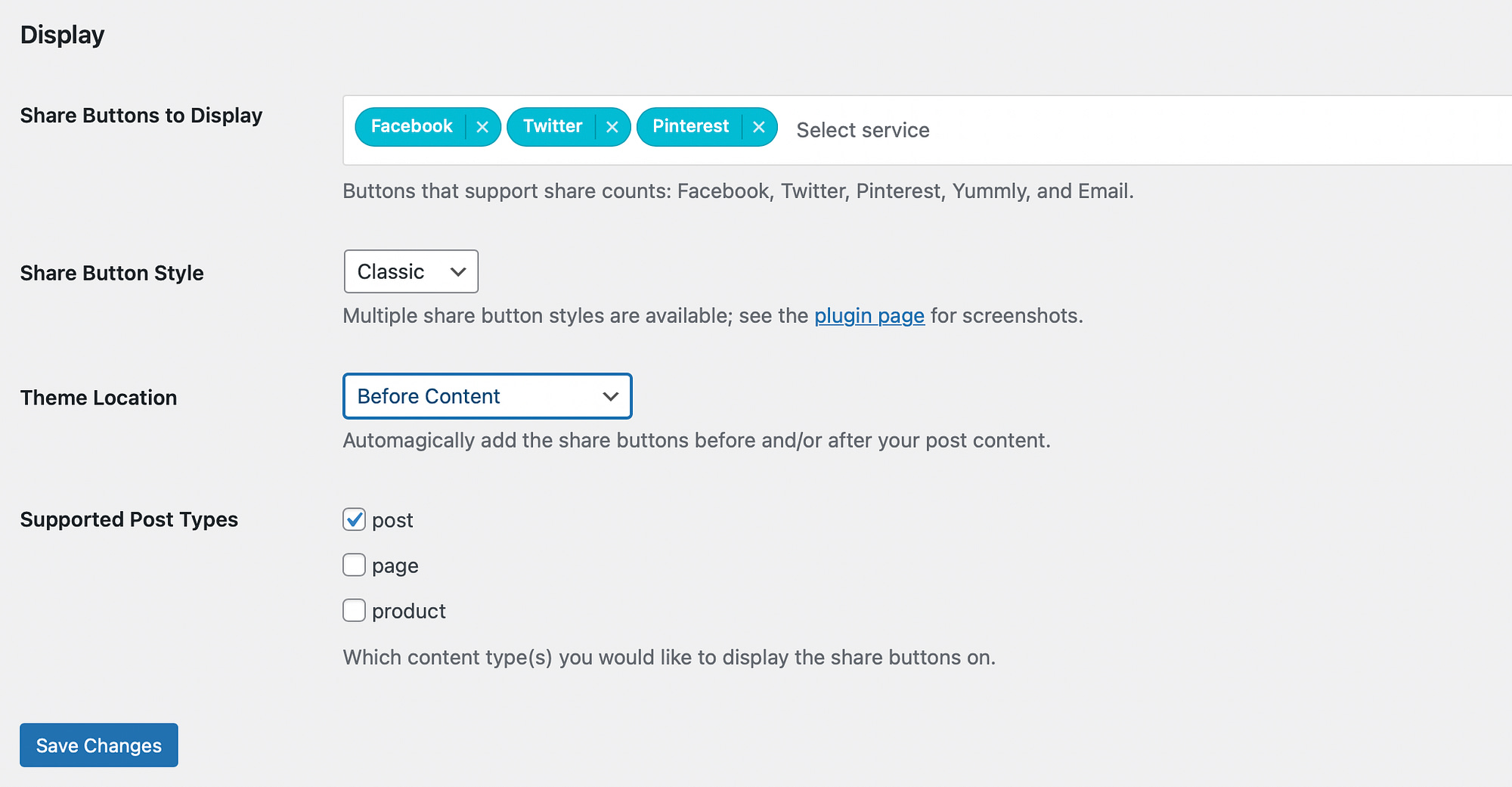The image is a horizontal rectangle displayed on a light gray computer monitor background. In the upper left corner, the word "Display" is written in black font. Beneath it, in slightly smaller black font, the text reads "Share buttons to display."

Adjacent to this on the right, a white rectangular area contains three horizontal turquoise ovals. Each oval features white text: the first oval reads "Facebook," with a white 'X' icon to its right; next is "Twitter," and finally "Pinterest". To the right of these ovals, inside the white bar, the text "Select service" appears in black font.

Below this section, the text "Buttons that support share counts: Facebook, Twitter, Pinterest, Yumly, and email" is listed. Moving back to the left column, bold black font displays the words "Share button style." Directly across from this, a horizontal rectangular area contains the word "Classic" with a downward arrow beside it.

Further down, the text "Multiple share button styles are available; see the plugin page for screenshots" features blue underlined font for the phrase "plugin page." The next section is labeled "Theme location" on the left, with a corresponding white horizontal rectangular area on the right, outlined in blue and containing the phrase "Before content" in blue font with a downward arrow.

Under this, the instruction "Automatically add the share buttons before and/or after your post content" is provided. Continuing in the left column, the text "Supported post types" is stated, followed by three options with checkboxes: "Post," "Page," and "Product." The "Post" option is selected with a turquoise checkmark.

Beneath "Product," the question "Which content types would you like to display the share buttons on?" appears in parentheses. At the bottom left-hand corner, a turquoise horizontal box with white font displays the words "Save changes."